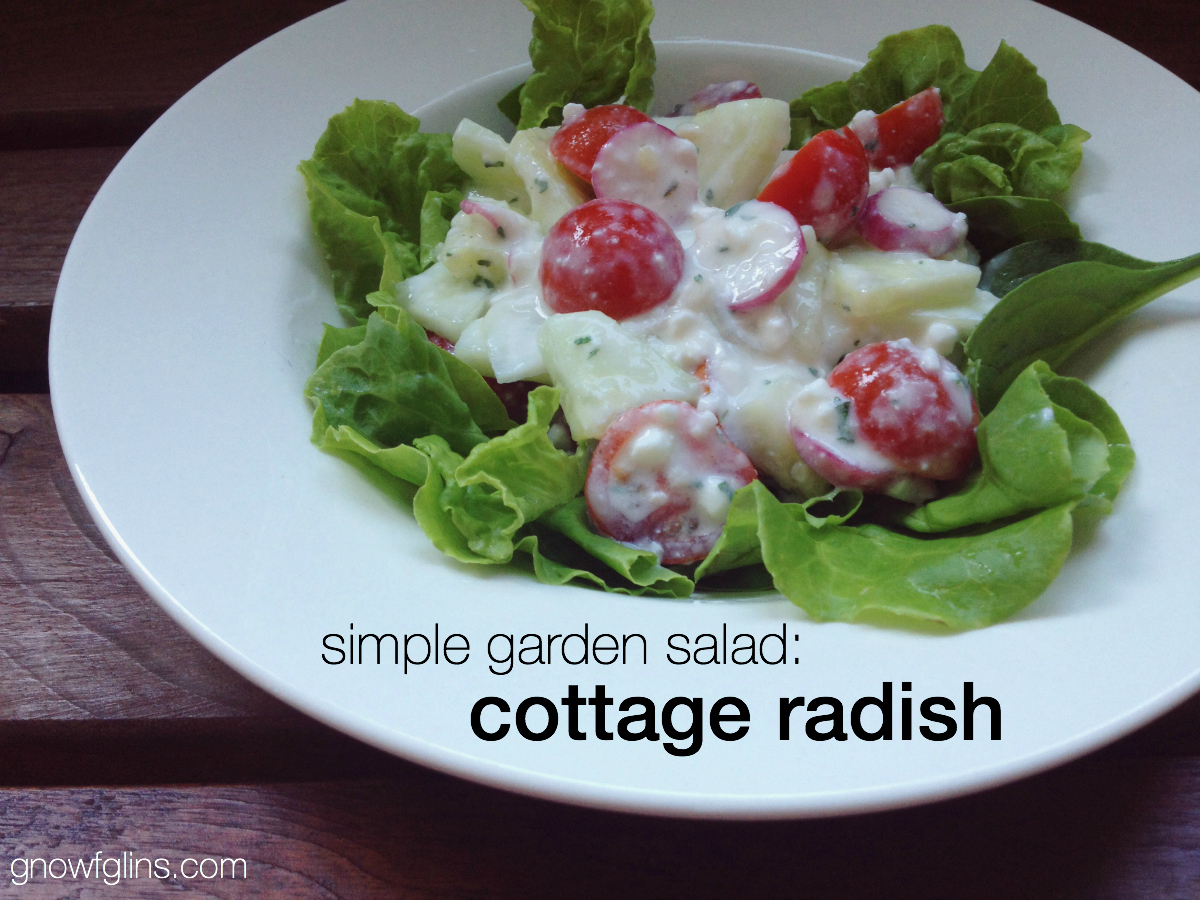This color photograph features a detailed image of a salad presented on a white dinner plate set on a dark, slatted wooden table. The salad comprises an abundance of pale green lettuce leaves, which appear to be romaine, mixed with sliced cherry tomatoes and finely chopped white radishes. The ingredients are generously topped with a creamy, herb-infused dressing, contributing to the salad's fresh and appetizing appearance. In the image, black text positioned in the upper center reads, "Simple Garden Salad: Cottage Radish," confirming the presence of radishes. Additionally, in small white text at the lower left corner of the photograph, the website "G-N-O-W-F-G-L-I-N-S dot com" is displayed.